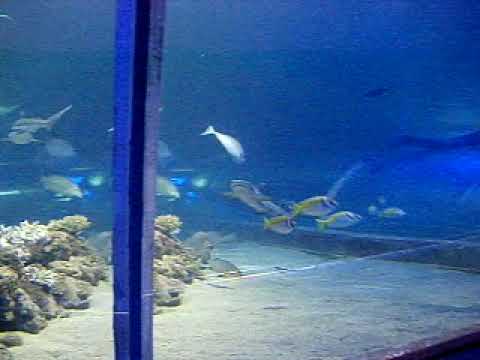This photograph captures the enchanting interior of an aquarium tunnel, where visitors can walk through and be surrounded by aquatic life from every angle. The tunnel is designed with blue-painted walls and floors, enhancing the underwater illusion. The glass arched above and alongside the walkway immerses visitors in a panoramic view of water, faux rocks, and corals. In the midsection of the tunnel stands a young man, possibly of Asian descent, sporting black hair, a white shirt, and light-colored pants, with his arms crossed. He appears to be facing back, engrossed in his surroundings. Behind him, distant figures of other visitors are visible, though their details are indistinct due to the image's pixelated quality. The setting is brightly lit, emphasizing the vibrant and captivating under-the-sea ambiance.